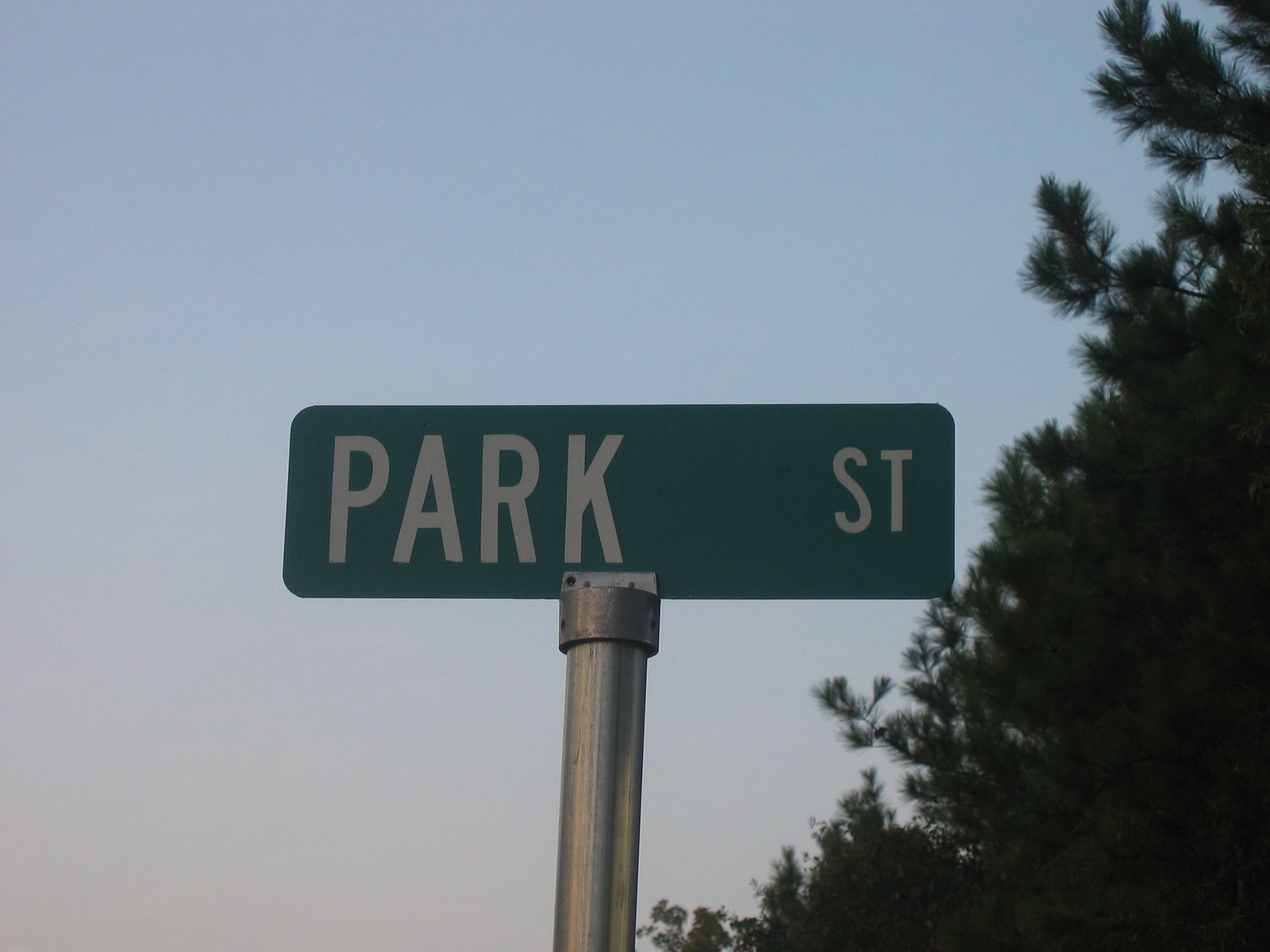This color photograph features a prominent rectangular street sign reading "Park Street" in bold white letters set against a green background, mounted at the top of a silver pole. The sign is centrally positioned in the image. To its right and extending diagonally upward towards the left is a lush, dark green pine tree, its dense foliage framing part of the sign. The backdrop consists of a softly graduated sky, transitioning from a light tan-brown hue at the horizon to a muted, hazy blue as it ascends, suggesting an overcast or possibly foggy day with some pollution affecting the clarity of the blue sky.